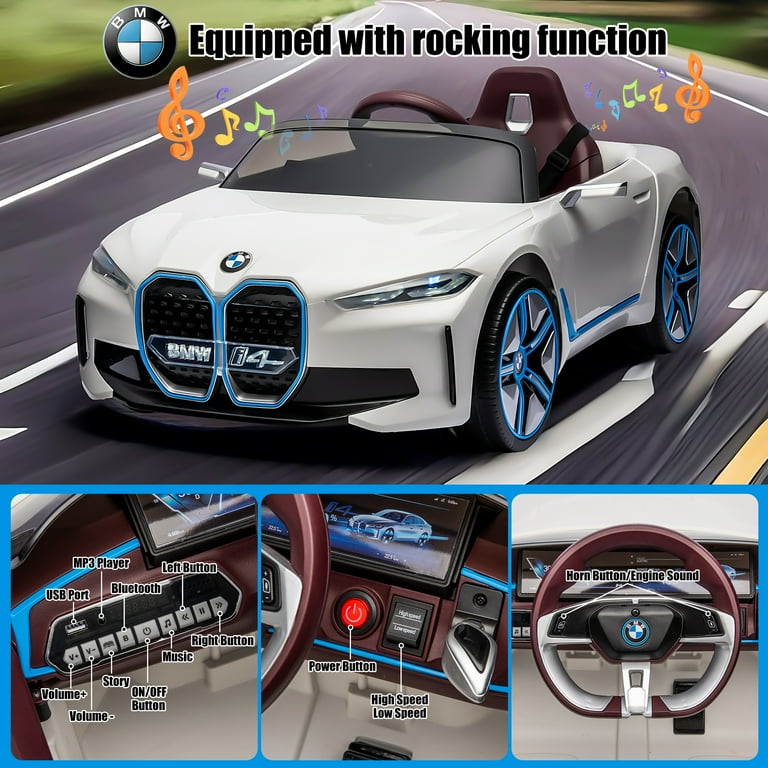The promotional image vividly details a child-sized, ride-in BMW i4 toy car, designed for young children aged 3 to 4 years old. The top section of the image prominently features a sleek, white BMW i4 model with the iconic BMW badge on the bonnet. The text "equipped with rocking function" is displayed at the top, while music notes and icons indicating various music features emanate from the car, suggesting its ability to play music. The lower part of the image is divided into three smaller panels showcasing the intricate interior details, such as the horn button, a power button, USB port, Bluetooth connectivity, story button, mp3 player button, volume control, and on/off button. The design of the image, employing CGI elements, clearly emphasizes the extensive features of the toy car, indicating it is a specialized promotional material to attract potential buyers.